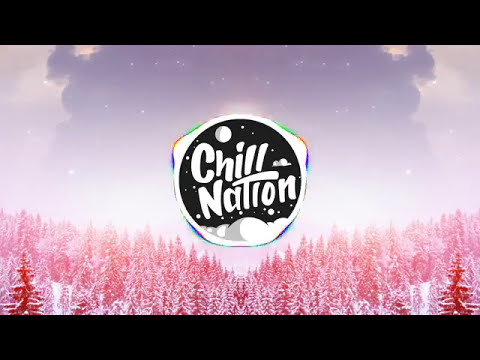The image features a prominently centered circular logo with the text "Chill Nation" in white font set against a black background. Outlining the black circle is a subtle pattern accented with rainbow colors, specifically green, orange, and blue. At the top of the circle sits a solitary white ball, while several smaller white balls adorn the bottom. The background behind the logo is predominantly grey and blurry, with grey clouds mimicking an arch-like structure. Beneath the logo, there's an expansive forest of towering evergreen trees, intriguingly colored in shades of red and pink, as if dusted with snow. Here and there, stars dot the sky, adding a touch of whimsy to the scene.